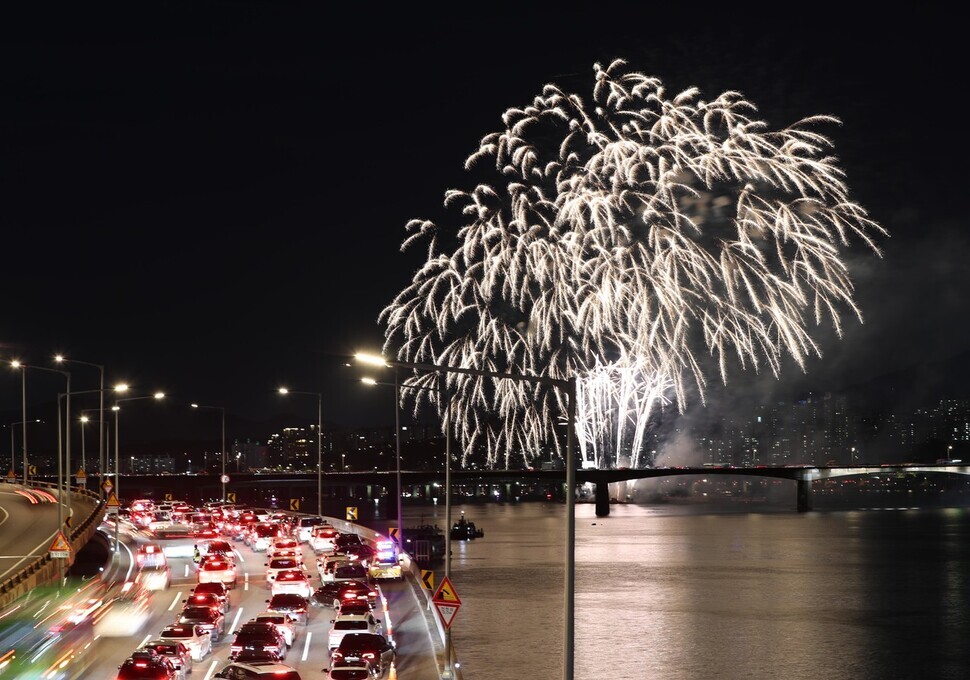The image captures a dynamic night scene with a highway teeming with traffic on the left-hand side, extending into a distant cityscape faintly illuminated by the lights of various office buildings. To the right, a river flows, crossed by a bridge in the mid-distance, where a barge or vessel appears to be the source of a fireworks display. The sky is pitch black, devoid of stars, likely due to the brightness from the fireworks and the glow from the vehicle lights. The image is partially black and white with some color correction, making it appear almost artistic in nature. The street lights predominantly cast a glow over the highway, and the cars are highlighted in red, enhancing the visual contrast against the monochromatic backdrop. A tall fence separates the highway from the river, emphasizing the division between the bustling roadway and the tranquil water. The fireworks bursting in white tones, lack vibrant hues, adding a nostalgic touch to the image. Overall, the picture offers a vivid portrayal of urban life at night, artistically enhanced to juxtapose the flowing traffic with the serene river and celebratory fireworks.